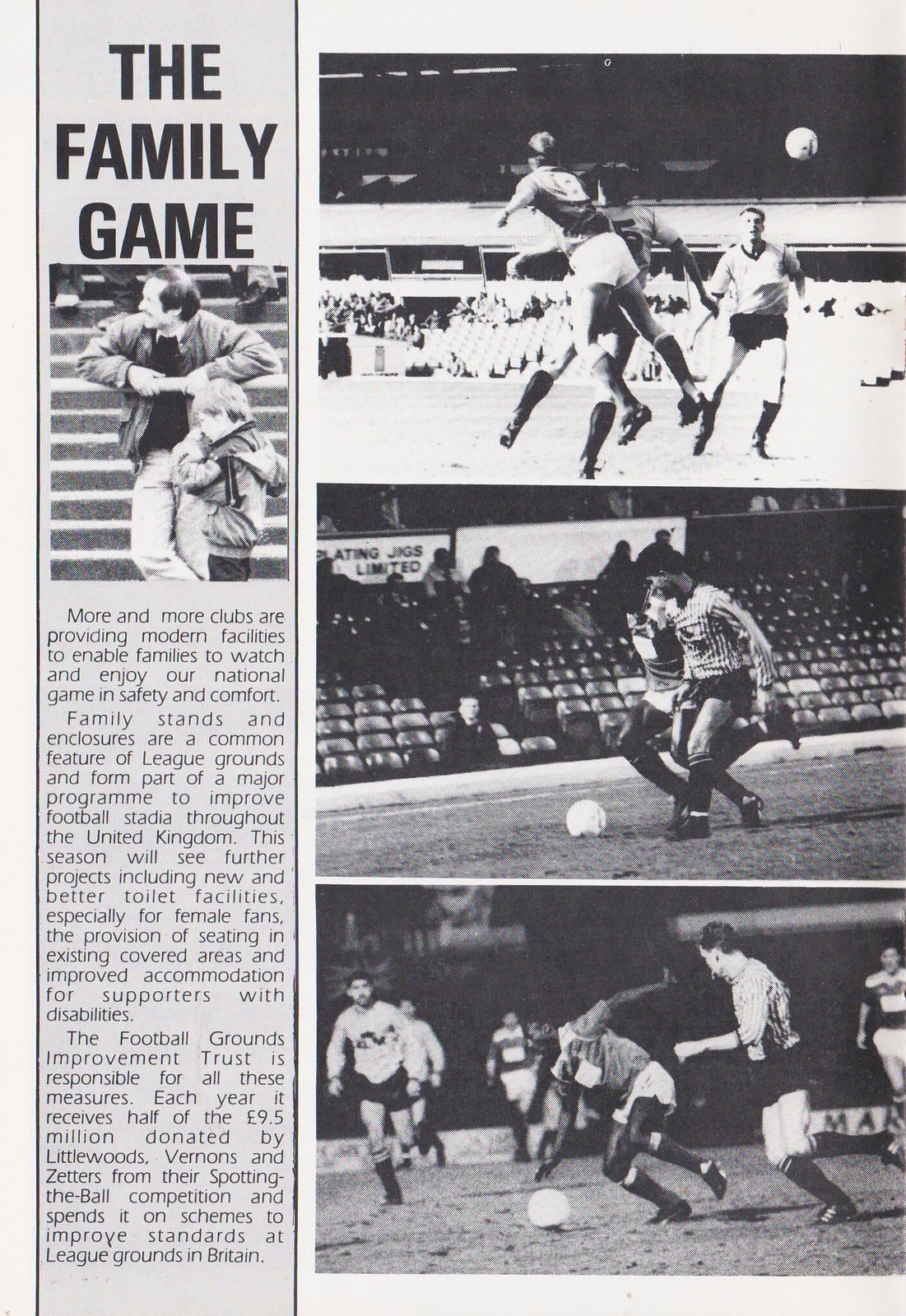A detailed photograph of a newspaper clipping titled "THE FAMILY GAME" in bold, black, all-capital sans serif font. The image is a monochrome collage, with the right two-thirds displaying three vertically stacked photographs. The bottom photograph shows soccer players seated around a ball. The middle image captures two players vying for ball control with sporadically filled stands in the background. The top photograph depicts two players attempting to head the ball, with another player in the distance and stands visible afar. On the top left, a father and son are shown enjoying a game from the stands, embodying the spirit of family attendance at soccer matches. The accompanying text discusses how more clubs are providing modern facilities, including new and improved toilet amenities, particularly for female fans, to enable families to watch and enjoy the national game in safety and comfort. This article highlights the ongoing efforts to modernize football stadiums throughout the United Kingdom to enhance the overall fan experience.